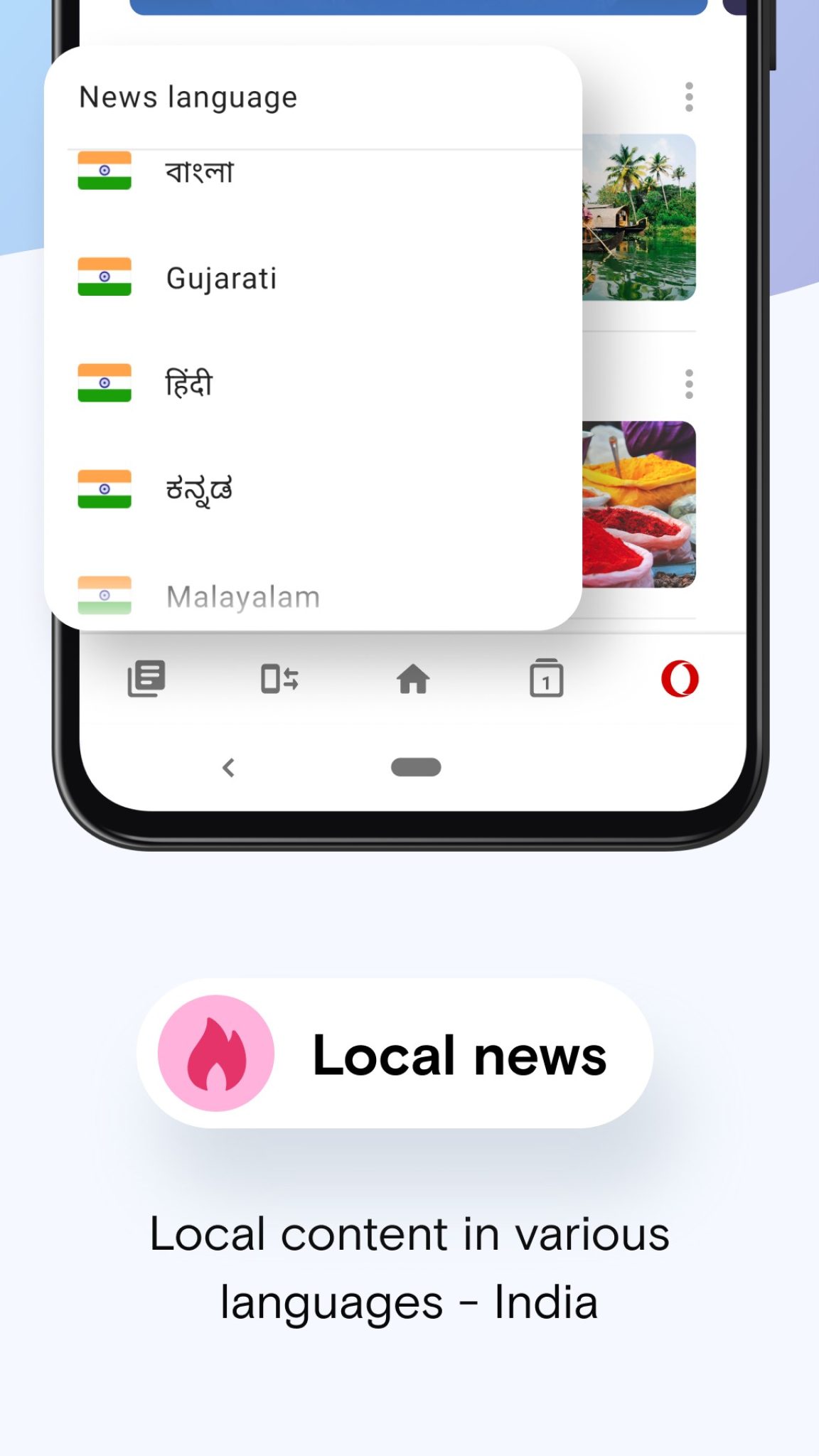In the image, we observe a mobile phone screen displaying a menu for language selection, which appears to belong to a news-related application or website. The interface prominently features the heading "News Language," under which various language options are listed in distinct scripts, suggesting a multilingual platform. Below this section, there is an entry labeled "Local News" with an apparent clickable link, indicating additional content. Further down, the text specifies "Local content in various languages - India," implying that users can choose their preferred language to access localized news content. This screenshot showcases the versatility of the application in catering to a diverse audience by offering news updates in multiple languages.